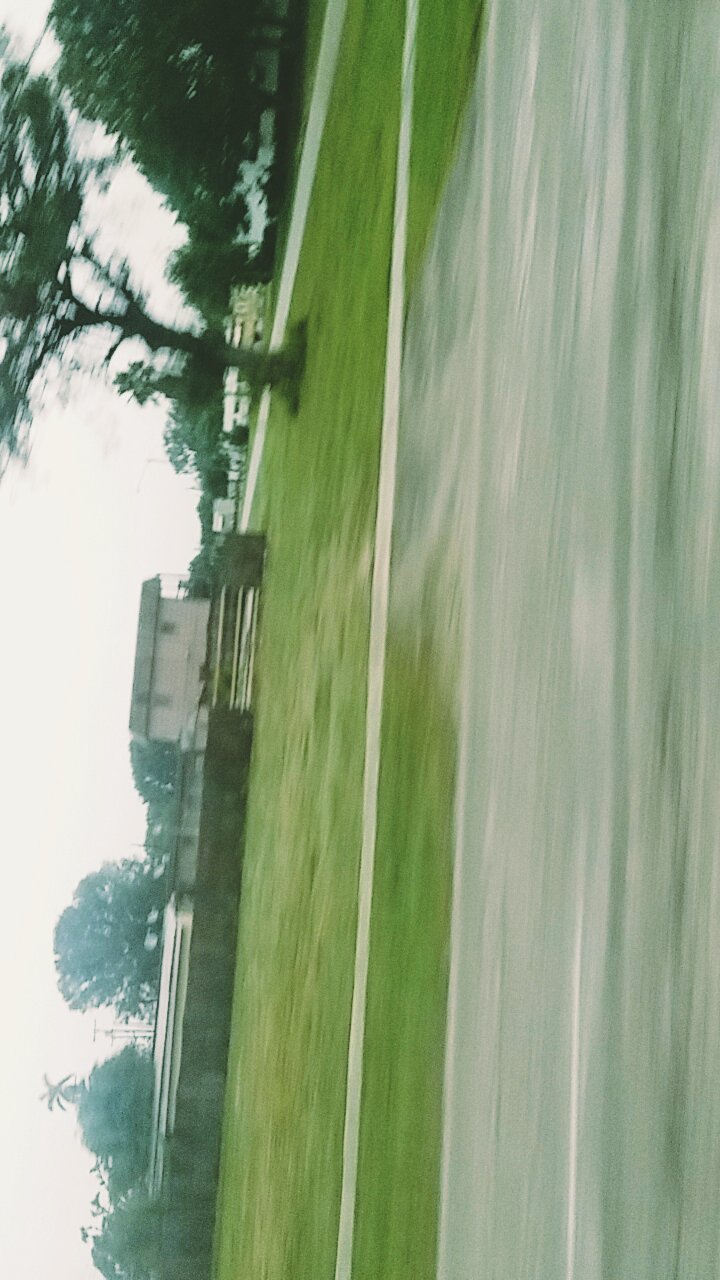The photo captures an outdoor scene, likely a yard, although the image is sideways and somewhat blurry. In the background, there are houses spread across a field, with a road in the foreground closest to the photographer. At the center of the image stands a white house with a gray roof, encircled by a brown fence. Adjacent to the house is a garage and a couple of trees, with their leafy tops visible above the structure. A distinctive palm tree is also noticeable in the distance. Power lines crisscross the sky, adding to the landscape's suburban feel. Between the house and the road, a tall tree with a sparse trunk and a dense canopy at the top reaches up to the skyline. Nearby, a smaller tree with a thinner trunk but a fuller spread of leaves adds to the natural scene.